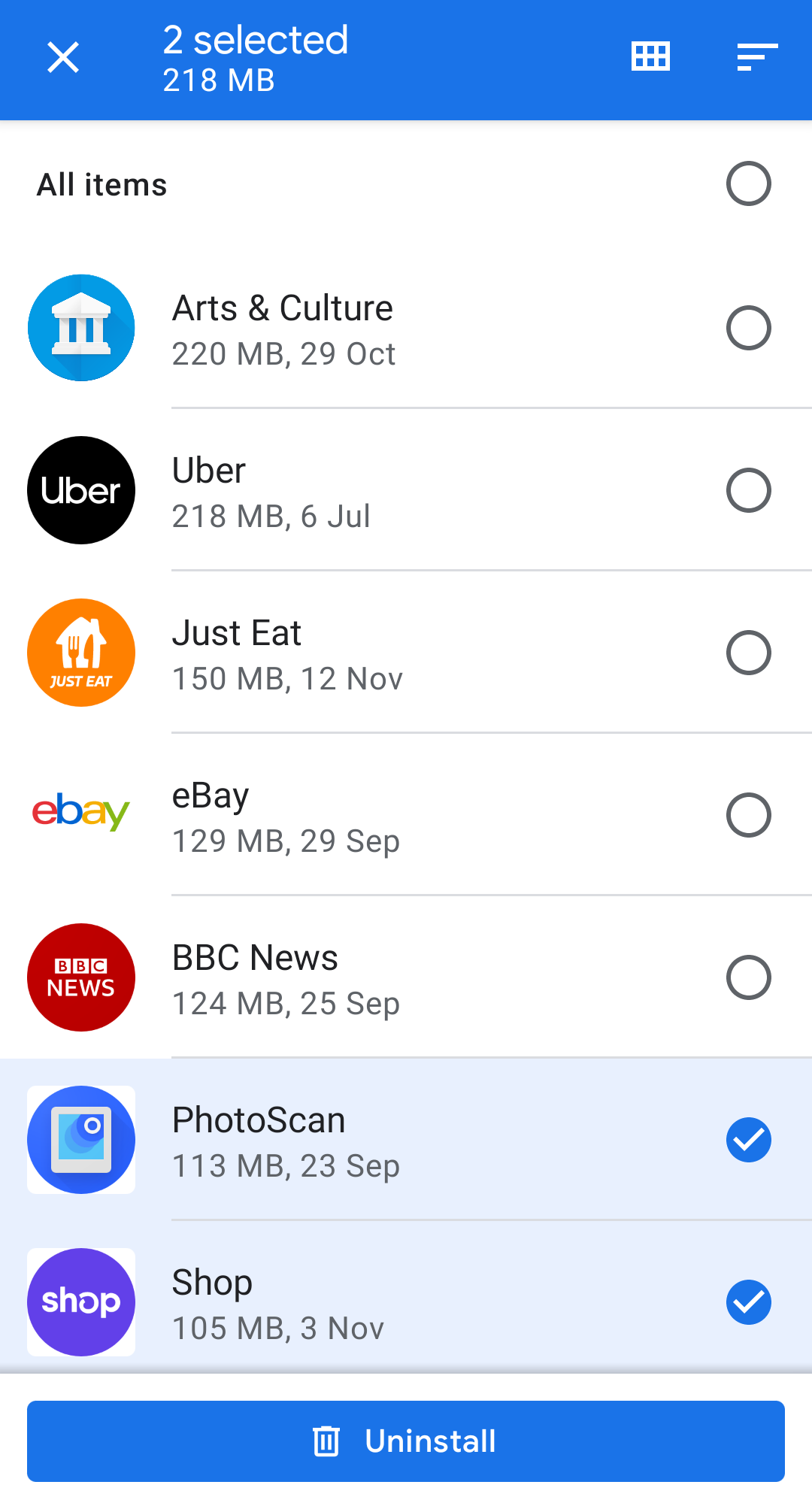The image displays a graphical interface with a blue header at the top. Within this header, there is an "X" button and text indicating "2 selected, 218 megabytes" in white. To the right, there are icons including a grid for item selection and a three-line menu.

Below the header, the interface lists various items organized in a vertical layout. Each item has a descriptive label, a specified file size in megabytes, and a date. Beside each item, there is an oval, some of which contain a blue background with a white checkmark. The items are as follows:

1. **Art and Culture**
   - File Size: 220 megabytes
   - Date: 29th of October
   - Selection Status: Not selected

2. **Uber**
   - File Size: 218 megabytes
   - Date: 6th of July
   - Selection Status: Not selected

3. **Just Eat**
   - File Size: 150 megabytes
   - Date: 12th of November
   - Selection Status: Not selected

4. **Ebay**
   - File Size: 129 megabytes
   - Date: 29th of September
   - Selection Status: Not selected

5. **BBC News**
   - File Size: 124 megabytes
   - Date: 25th of September
   - Selection Status: Not selected

6. **Photoscan**
   - File Size: 113 megabytes
   - Date: 23rd of September
   - Selection Status: Selected (indicated by a blue oval with a white checkmark)

7. **Shop**
   - File Size: 105 megabytes
   - Date: 3rd of November
   - Selection Status: Selected (indicated by a blue oval with a white checkmark)

At the top, there is the text "All items" in black. The interface is designed to allow the user to select various items, indicated by the blue checkmarked ovals.